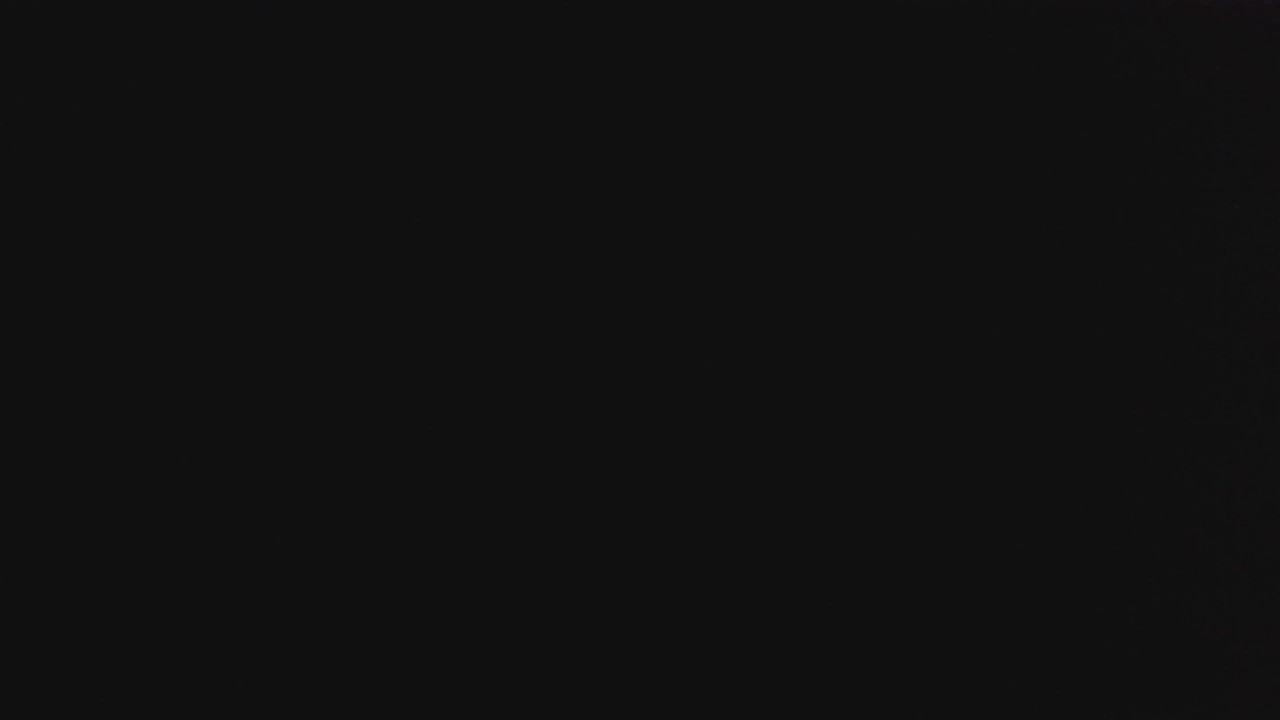The image displays a completely black rectangle, void of any discernible features, text, or identifiable elements. Resembling a blank canvas, it spans an approximately 16:9 aspect ratio, characteristic of widescreen dimensions. The stark blackness dominates the entire frame, leaving no room for interpretation or visual cues. This image's uniform darkness might be perceived as an error, but it could also be intentional, prompting the viewer to simply acknowledge its presence.